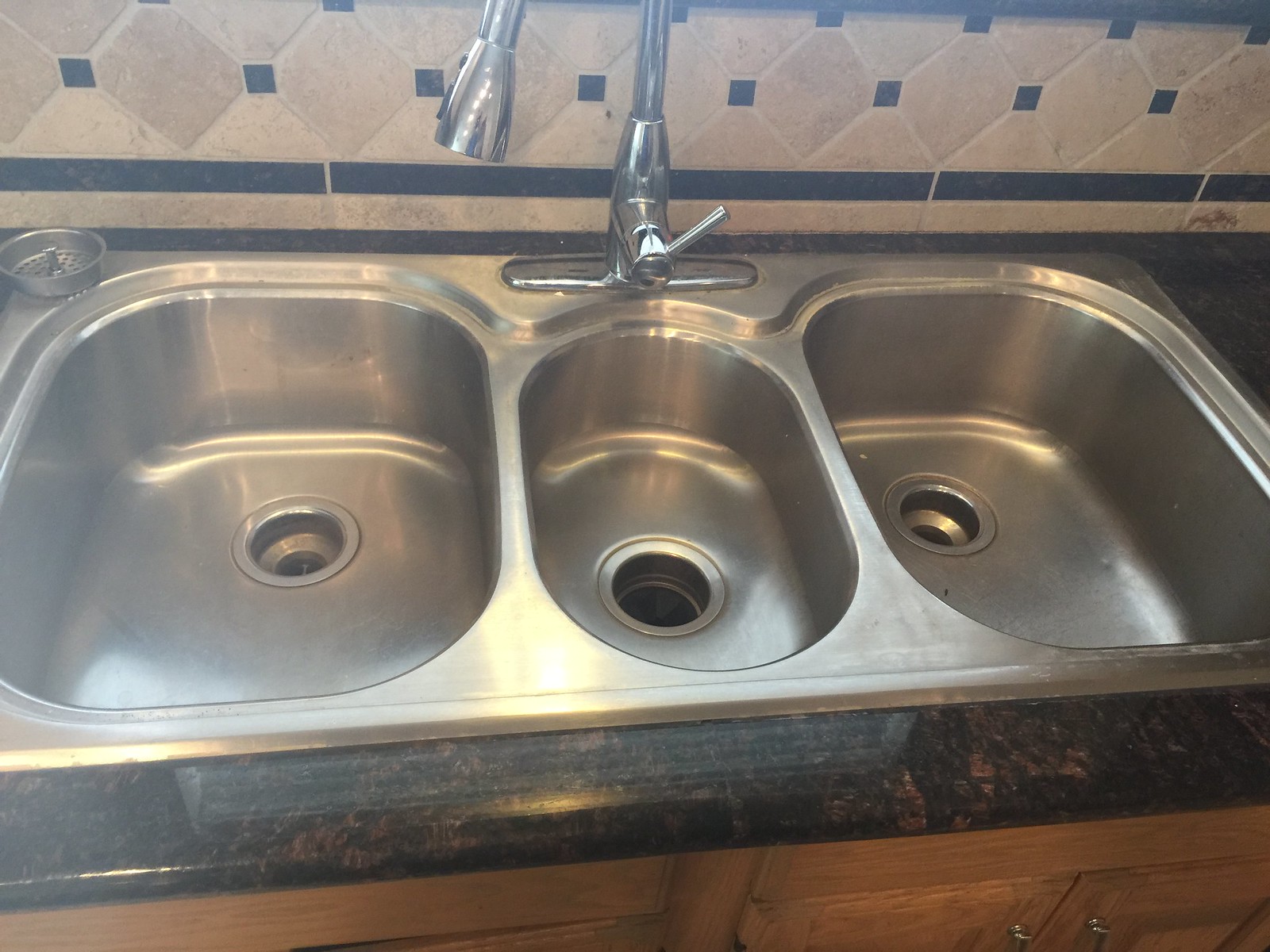This detailed photograph features a stainless steel sink with three distinct basins. The left and right basins are large and square, while the middle basin is smaller and oval in shape. Each section has a drain, with a strainer visible near the top of the left basin. The sink is mounted within a dark brown, possibly wooden, countertop, and flanked by oak cabinets underneath. Above the middle basin is a swan-shaped faucet adorned with two black buttons designed to switch between spray and stream modes. A single handle sticks straight up in front of this faucet, allowing for easy control. The backsplash is a striking mix of cream, very light tan, and white tiles arranged diagonally, accentuated by evenly spaced black squares forming two horizontal stripes near the bottom. The scene is immaculate and emphasizes the modern, functional design of the kitchen setup.